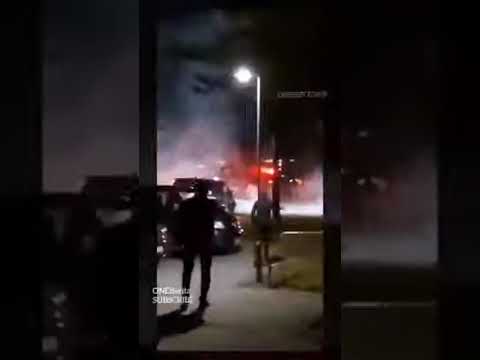The photograph shows a night-time city street scene framed by a large black border. It appears to be taken from a dark indoor area, looking out through either a doorway or a window. The main focus of the image is a streetlamp centrally located, illuminating a section of the scene. Directly under the streetlamp, a person is walking or standing, their shadow stretching out behind them due to the light's intensity. A small concrete walkway and a grassy area flank the scene to the right, while to the left, a black van and a few other cars are parked. Smoke or haze is visible in the background, suggesting either street activity or an emergency situation. Trees and shrubs are faintly discernible, blending into the night. In the distant background, vague spotlights imply a larger open area, possibly a parking lot. The bottom of the image contains text, possibly for a subscription prompt, though it is partially obscured and challenging to read.